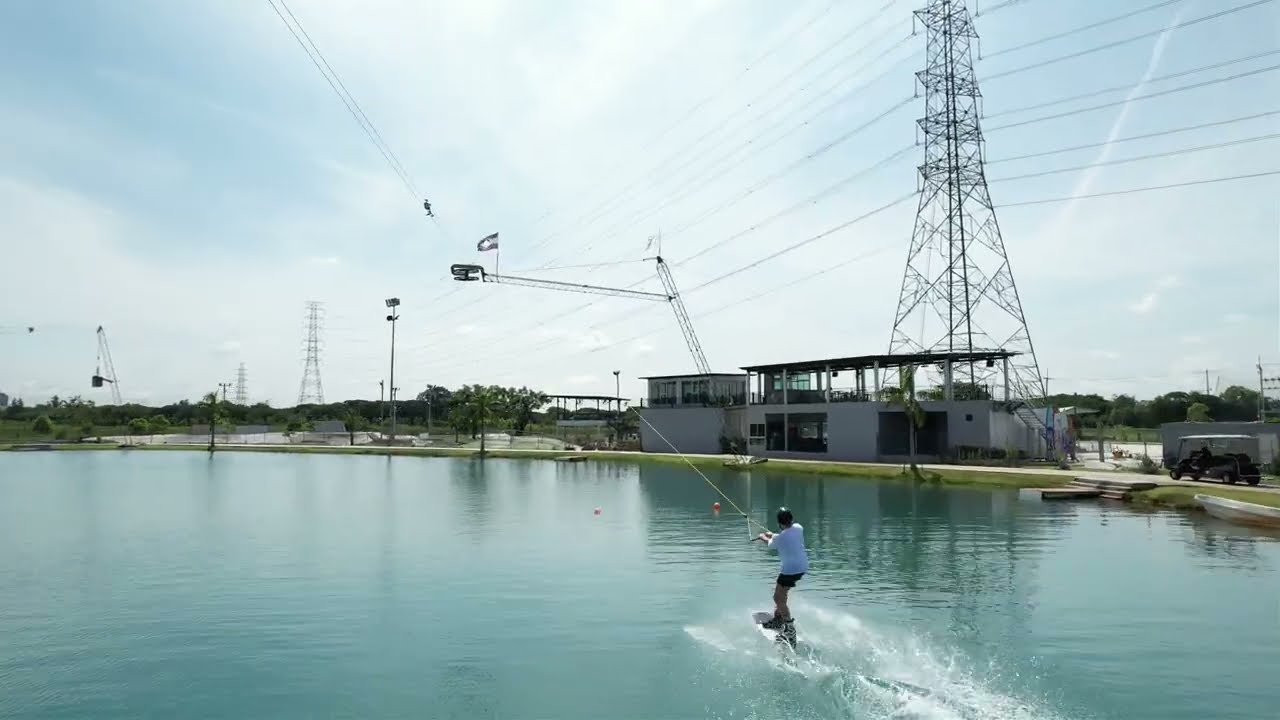The image captures a man engaged in a water sport, firmly standing on a snowboard-like board gliding over the surface of a calm, greenish-turquoise body of water, reminiscent of a man-made lake. He is gripping a handle connected to a thin white line that extends upward, though it's not clear what's creating the tension on the line pulling him forward. The water behind him is splashed, forming a trail. The setting includes a bank bordering the lake, featuring a mix of cement and grass areas. Buildings are visible on this bank, and in the background, multiple electrical towers stretch into the distance, interconnected with numerous wires. The sky above is a light blue, adorned with thin white clouds. Additionally, there's another person or figure seen higher in the sky, suggesting the presence of a suspended or descending activity, though its exact nature is indistinct. The overall scene merges elements of natural calmness with industrial touches, linking the serene water with structural surroundings.